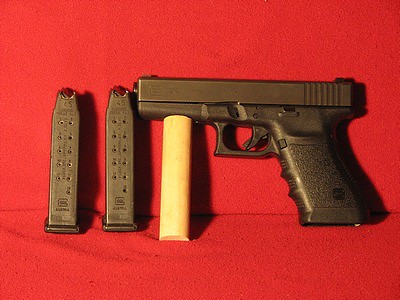This image features a small, black pistol, potentially a 9mm handgun, positioned against a rich red fabric backdrop. The gun is situated on this red cloth, which drapes both above and below it, and its sleek black body contrasts sharply with the background. The pistol includes standard features such as a trigger and a grip around the handle, with a visible slide on the top for chambering the next round. Notably, a light tan cylindrical block, potentially wooden, is placed beneath the barrel, propping the gun up.

To the left of the firearm, there are two magazines, each designed to hold ammunition, seemingly marked with "4.5" or ".45" on them. These dark brown or black magazines taper at the top and feature a series of small, possibly eleven, double holes starting just below the tapered section, presumably for visual or functional reasons. Each magazine also has a pronounced lip at the bottom, likely for easier handling and insertion.

Overall, the photograph captures these elements with intricate detail against the vivid red sheet, which appears folded near the end of the gun, adding texture to the scene.